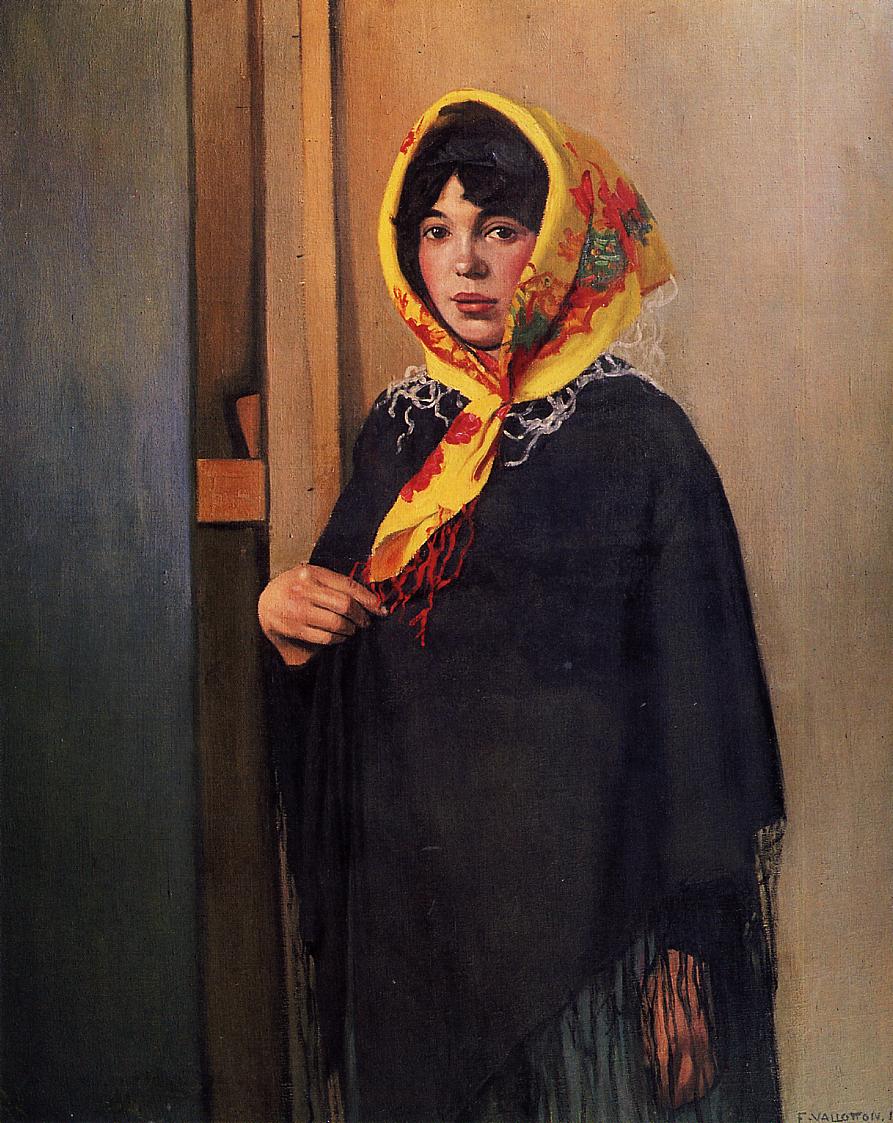This painting depicts a young woman with dark, black hair, adorned with a yellow scarf that features prominent red blotches and slight hints of green, intricately wrapped around her head and tied just beneath her chin like a kerchief. She exudes a melancholic air, her sad eyes hinting that she may have been crying, contrasting with her attractive appearance and very red, full lips. She is clad in a black poncho or cloak-like garment, which drapes her body fully except for her right arm. Her right hand is raised, her index finger pointed towards her chest, accentuating her introspective demeanor, while her left arm hangs down by her side, barely visible. The backdrop is composed of a wooden wall, lending a rustic atmosphere, or possibly a brown doorway, suggesting she stands at the threshold of a room. The detailed textures and colors of her attire and the nuanced emotion in her expression are beautifully captured in this poignant artwork.